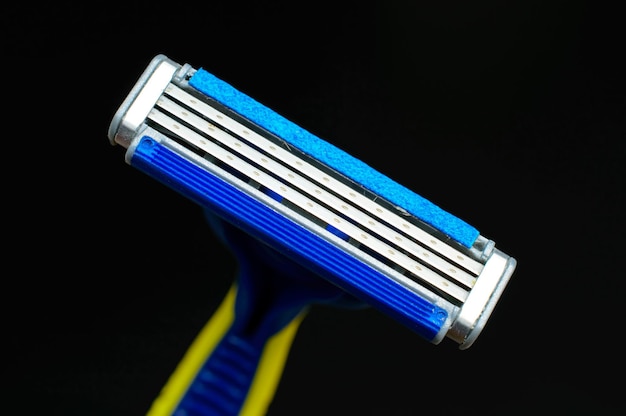This close-up image features a manual safety razor, set against a completely black background. The razor is positioned diagonally, drawing attention to its functional elements. It flaunts a triple blade system, with three sharp metal blades encased between a turquoise, presumably moisturizing, strip at the top and a ribbed turquoise comfort strip at the bottom. The peripheries of the blade section are framed with silver and grey borders on both the left and right sides. The handle of the razor is designed for grip and ease of use, featuring a blue central strip with yellow plastic sides. The overall design suggests a blend of functionality and comfort, likely a product from Galette, aligning with its characteristic color scheme and design elements.